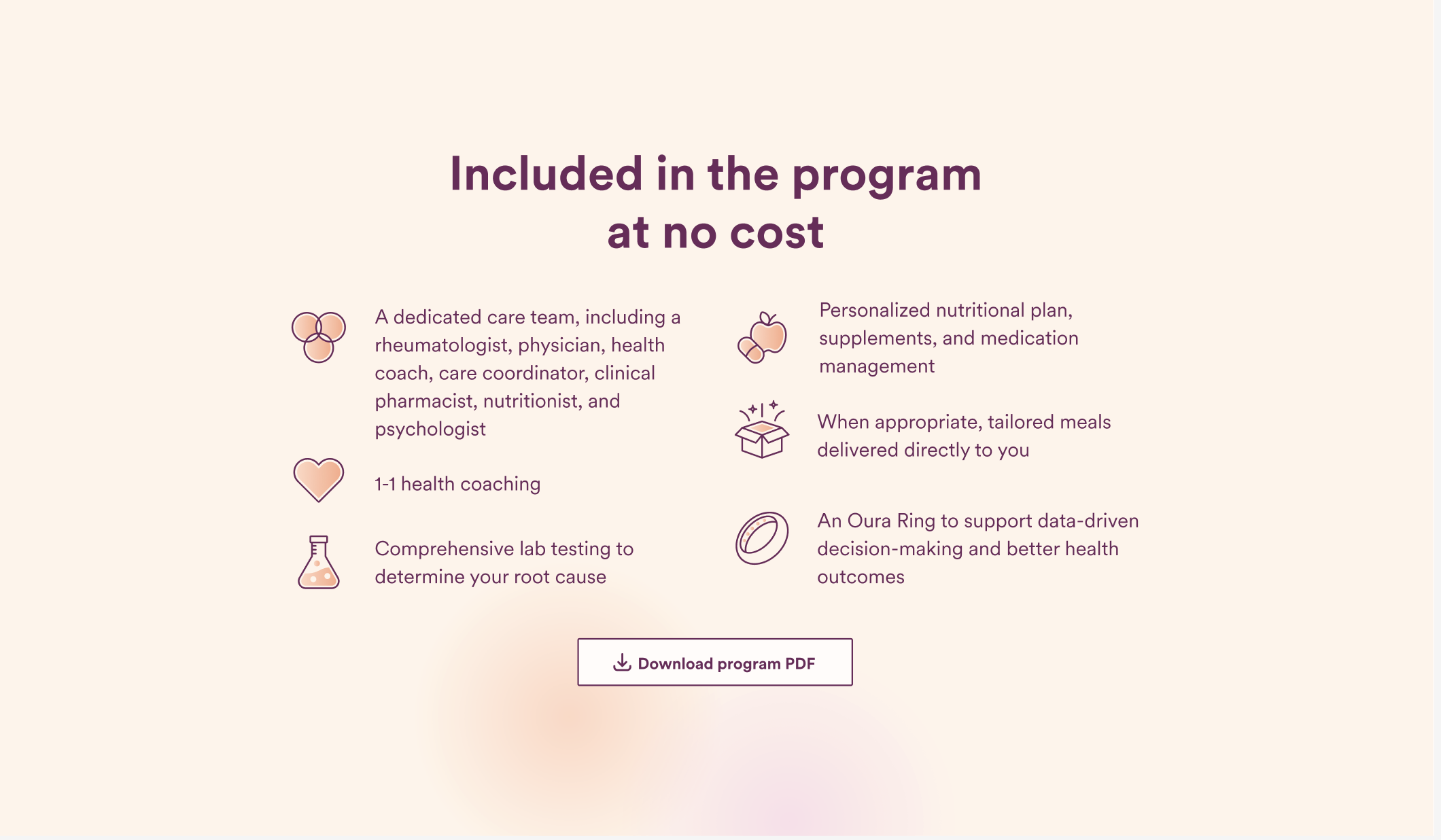The image features a predominantly pink background, with a multitude of informational elements included at no cost. At the center, there is a pink square with purple text explaining the offerings of the program. Surrounding the square, three concentric circles highlight the comprehensive care provided by a dedicated team, which includes a rheumatologist, physician, health coach, care coordinator, clinical pharmacist, nutritionist, and psychologist.

In one section of the image, there is mention of "one-to-one health coaching," "comprehensive lab testing to determine your root cause," and a "personalized nutrition plan" that incorporates supplements, medication, and management. An open box icon suggests that these elements are tailor-made and delivered directly to the participant.

A surrounding ring emphasizes the program's focus on data-driven decision making for better health outcomes. Additionally, there is a rectangle with an arrow pointing downwards indicating the option to "download program PDF."

Overall, the image includes six distinct icons representing various aspects of the program, indicating its all-encompassing approach to health and wellness.